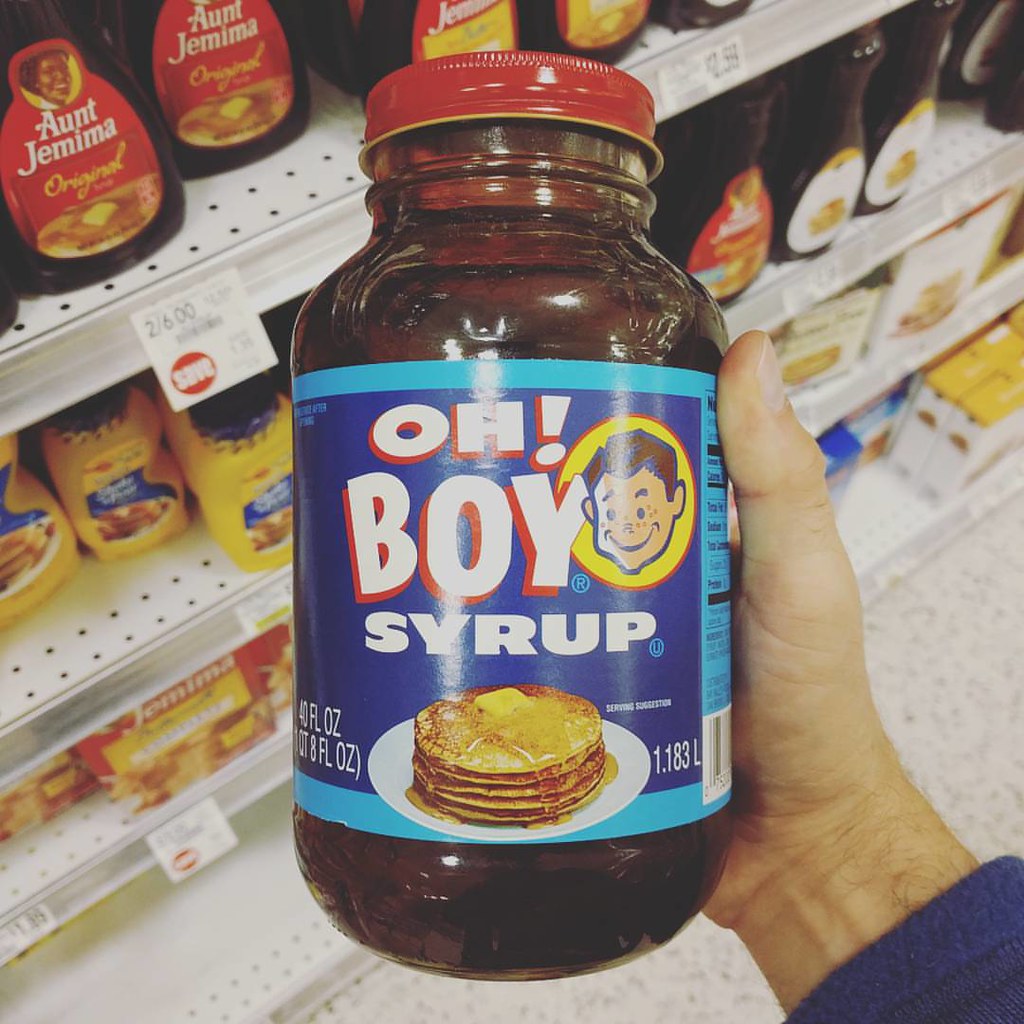In this detailed photo taken in a grocery store, a right hand with a fair complexion, wearing a long-sleeved blue shirt, is holding up a glass bottle of "Oh Boy Syrup" prominently in the center of the image. This bottle features a red lid, a distinctive light and dark blue label bordered in red, and large white text that reads "OH BOY Syrup." The label also includes a yellow circle with a cartoon image of a 1950s-style boy with black hair and a smiling face, alongside a depiction of a white plate with a tall stack of pancakes topped with butter and syrup. The background reveals white peg shelves with four visible layers filled with various brands of syrup and boxes of pancake mix, including Aunt Jemima syrup and Shake and Bake pancake mix. The shelves have distinctive circular holes drilled in pairs. Price tags indicate two for six dollars on Aunt Jemima syrup and $2.59 on an adjacent item. The floor beneath is white tile with gray specks. On the top left corner, the familiar red-labeled Aunt Jemima syrup bottle can be seen. The entire setting and product arrangement suggest a well-stocked and organized grocery aisle, with the syrup bottle being examined from a first-person point of view.